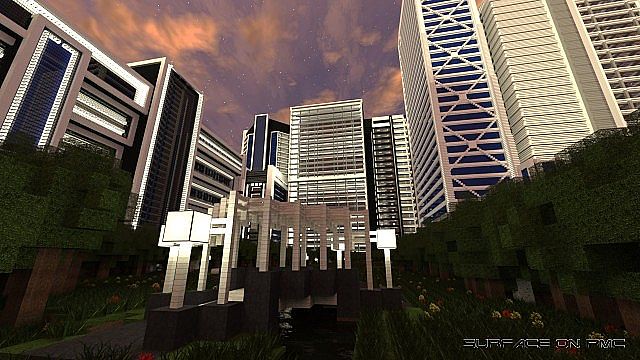This image depicts a stunning urban area created using the UrbanCraft resource pack, often associated with the game Minecraft. The scene captures a meticulously designed modern cityscape during what appears to be twilight, with a sky painted in hues of purple and orange and dotted with some white stars. Dominating the skyline are several high-rise buildings showcasing contemporary architecture. 

On the left, there's a five or six-story rectangular building adorned with sections of brownish-copper, black, and white, while the right side features a much taller structure, possibly 30 to 50 stories high, characterized by a crisscross pattern and primarily white coloring with some black accents, giving an impression akin to a hotel or corporate office. The middle of the scene features another towering building with multiple rooms and windows, demonstrating an urban design sense with a modern sculpture, outdoor lights, and trees dotting the courtyard below.

In the bottom right corner of the image, there is a watermark with the text "SURFACEONPMC," subtly acknowledging the creator. The courtyard, forming a U shape with the surrounding buildings, appears slightly obscured by darkness, but reveals elements such as hedges, a garden area, and unique lighting structures with white cubes atop poles. The entire landscape, bathed in ambient lights, combines to create an urban design that is both highly detailed and visually captivating, all constructed within the pixelated realm of Minecraft.